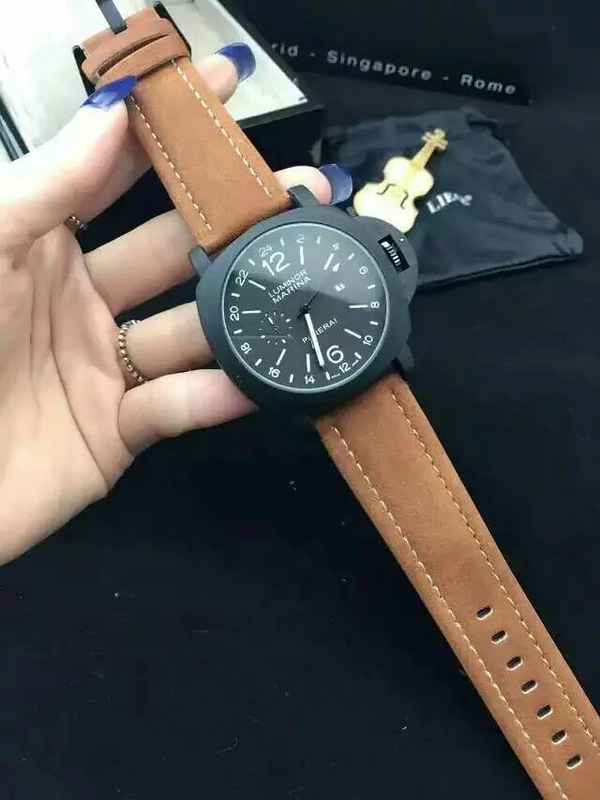This photograph, oriented with its long side stretching from top to bottom, captures a detailed close-up of a person's hand holding a sophisticated wristwatch. The watch, with a sleek black design contrasted by white hour markers and numerals, prominently displays the label "Luminor Marina" at its center. Notably, the watch face offers dual time measurement, featuring both a 12-hour clock and a 24-hour clock format. A subtle spinning wheel is located on the right-hand side of the watch face.

The watch is fastened with a brown band, intricately stitched and punctuated with adjustment holes on its lower half, designed to secure the watch comfortably on a wrist. The person holding the watch has their palm facing upwards, revealing blue nail polish and wearing rings on both the forefinger and ring finger, adding a touch of personal style to the image.

The background of the image transitions from a solid black at the bottom to a slightly revealed accessory—a bag adorned with a small, golden violin—providing a refined and harmonious backdrop to the main subject.